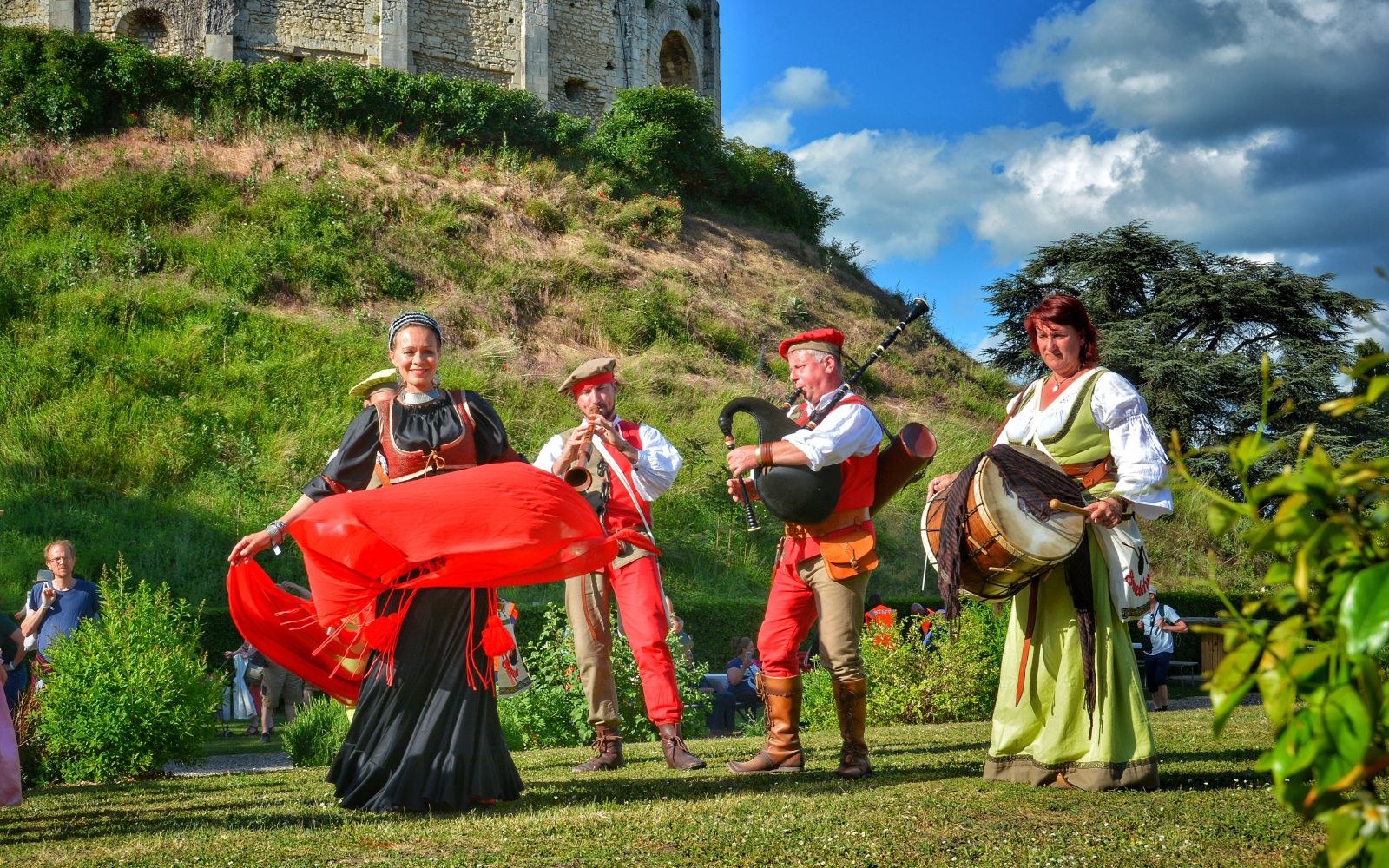This outdoor photograph captures a lively Renaissance fair scene set on a grassy hill under a bright blue sky dotted with white and gray clouds. In the foreground, four performers in vivid period costumes are engaging the audience. On the left, a woman in a black dress with ruffles, paired with a red vest, dances with a large red scarf swirling around her. Next to her, a man with a beard plays a trumpet-like horn; he is dressed in a distinctive jester-like outfit featuring a white long-sleeved shirt, a red and tan vest, and pants split into red and brown halves. Beside him stands another man similarly attired, playing the bagpipes. On the right, a woman clad in an olive green dress with white bell sleeves and a white collar strikes a large mounted drum with a drumstick. Behind the performers, a grassy hill slopes upwards, revealing a partial stone wall of a castle at its peak. In the background, a scattering of onlookers can be seen, enjoying the performances on this sunny day.